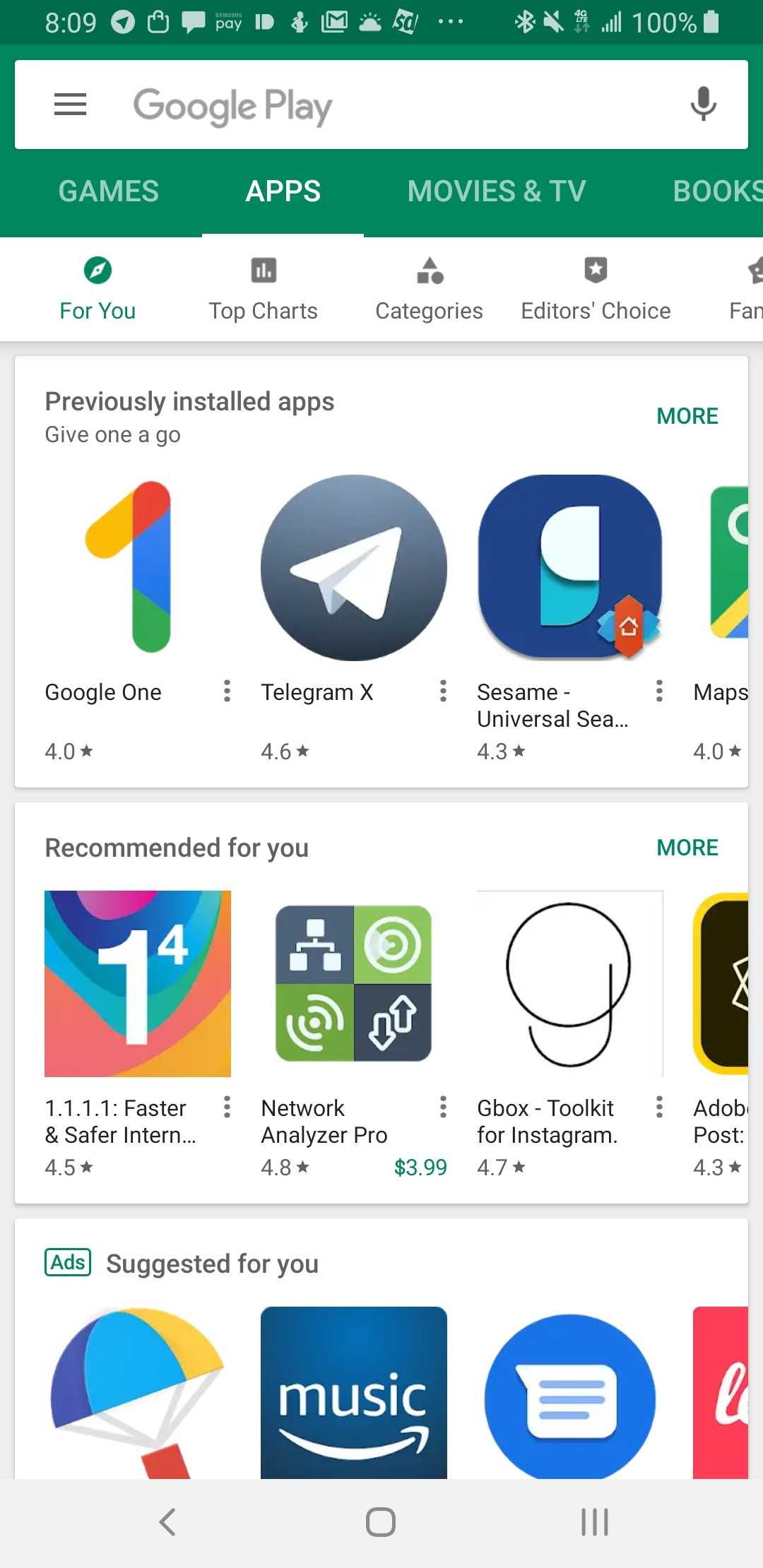The image depicts a screen from the Google Play app store. 

At the very top, the screen shows the current time as 8:09 on the left-hand side. To the right, a series of status icons are displayed, including a Bluetooth icon, a mute connection icon, and a battery icon indicating a full 100% charge.

Below this status bar, the "Google Play" logo is prominently displayed in gray text on the top left of the screen, next to a white search bar featuring a microphone icon on the right side for voice search functionalities. 

The navigation bar underneath the search bar includes four categories from left to right: Games, Apps (which is currently selected), Movies & TV, and Books (though only part of the Books category, "Book," is visible due to cropping of the image).

Beneath the navigation bar lies another row of categories. These include: "For You," "Top Charts," "Categories," "Editor's Choice," and one more category that is cut off and thus not visible in the image.

The next section is labeled "Previously Installed Apps" and lists a few apps including Google One, Telegram X, Sesame Universal, and Maps, against a white background.

Following this section is "Recommended For You" displaying several apps: "1.1.1.1: Faster & Safer Internet," "Network Analyzer Pro," "G-Box Toolkit," and Adobe. 

Finally, at the bottom of the screen is a "Suggested For You" section displaying partially visible app icons. The visible icons include a colorful animated parachute with indigo blue, light blue, and yellow hues, a music app shown as a blue square with "Music" written in white and accompanied by a white curved line, and another blue circle icon with a message bubble on it. Part of a red app icon is also visible on the far right.